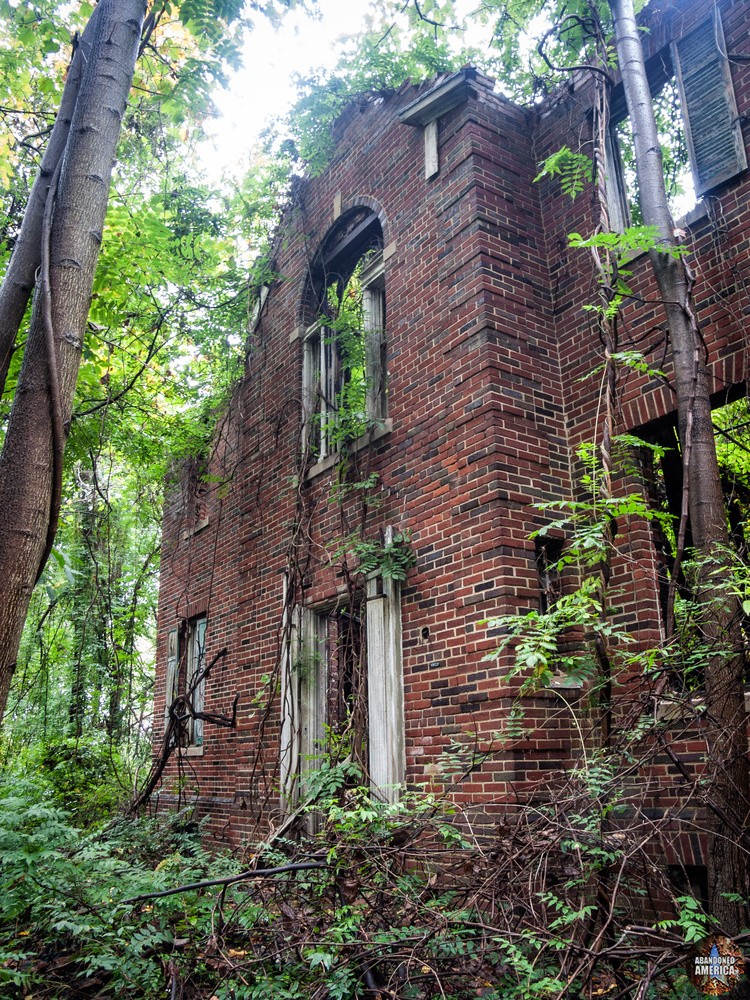This photograph captures the haunting beauty of an abandoned two-story red brick building that has clearly seen better days. The once majestic structure is now enveloped by nature. Vines creep up the exterior walls and encircle the building, while missing sections of the walls reveal glimpses of the dilapidated interior. The remnants of a shattered window and a non-existent door allow the viewer to peer inside, where trees and dense foliage have taken root, reclaiming the space. Tall green trees soar around the house, indicating that the picture was taken during the height of summer when vegetation is in full bloom. The porch steps have vanished, and the remaining wooden elements, including the window frames and shutters, are rotten and decayed. What was once a beautiful home is now an overgrown relic, cloaked in weeds, leaves, and the relentless grip of time.